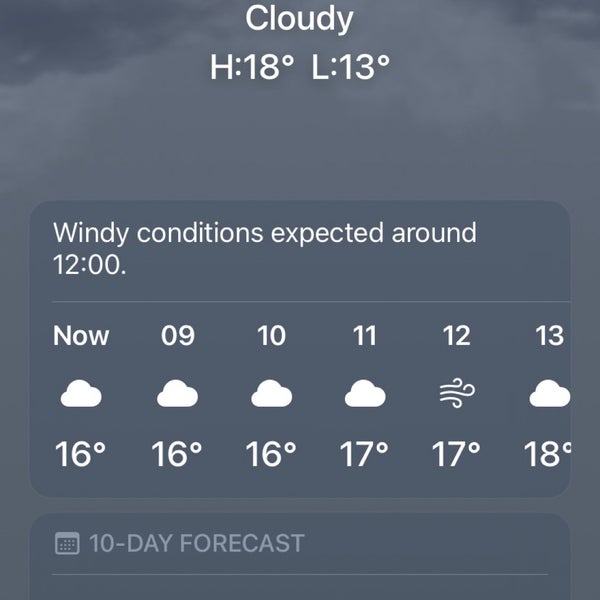Screenshot Description of Weather App Display: 

The screenshot portrays a segment of a weather application with a light gray background adorned with subtle cloud shapes. At the very top-center, the app displays white text that reads "Cloudy." Just below this, it provides the temperature details: "H: 18°C, L: 13°C."

Beneath this text, a pale blue rectangle with curved edges appears. The top portion of this rectangle is slightly darker blue. At the top of this rectangle, in white text, it reads "Windy conditions expected around 12 o'clock." 

Below this informative note, on the bottom of the rectangle, a series of icons indicates the expected weather. From left to right, there are four cloud icons followed by a windy icon and another cloud icon.

Further detailing the hourly forecast:
- A horizontal timeline is presented with labels: "Now, 09, 10, 11, 12, 13."
- Directly below these time markers, the respective temperatures are shown: "16°C, 16°C, 16°C, 17°C, 17°C, 18°C."

At the very bottom of the image, the top portion of another dark, pale blue rectangle is visible. The upper left corner of this rectangle features a calendar icon accompanied by light gray text that reads "10 Day Forecast." This section is underlined with a thin horizontal line extending from left to right.

Summarizing the weather forecast: The weather app indicates a cloudy day with a high of 18°C and a low of 13°C. Windy conditions are expected around noon, with a temperature of 17°C anticipated at that time.